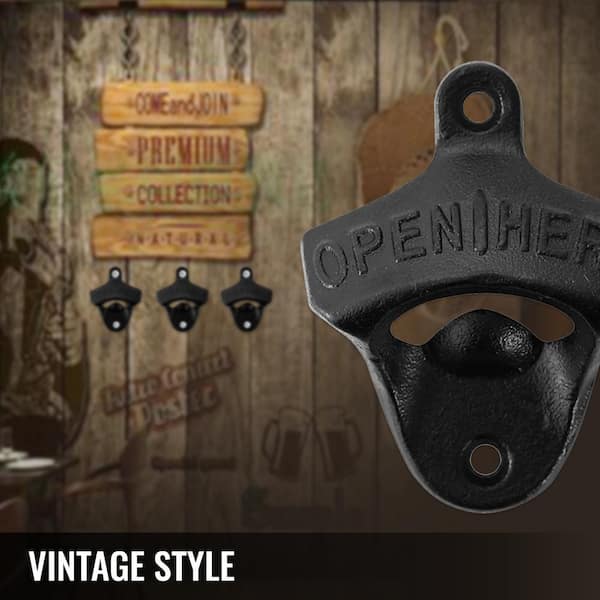The image showcases a weathered wooden wall adorned with various vintage-inspired elements. At the bottom of the image, a black banner with white font reads "vintage style." On the right side of the wall, there is an antique-style bottle opener made of black-painted iron, featuring the engraving "open here." This opener has mounting holes at the top and bottom. To the left of this opener, an image of two beer mugs is visible. Additionally, three more identical bottle openers are displayed further left on the wall, replicated to appear as though they are part of the background, though they are more sharply defined.

Above these openers, four wooden signs with a lighter, yellowish hue contrast the aged wood background. These signs read, from top to bottom: "come and join," "premium," "collection," and a smaller, less legible text that appears to say "natural." The wood panels behind these elements are vertically aligned and exhibit a rustic, somewhat blurry appearance, enhancing the image's vintage aesthetic.